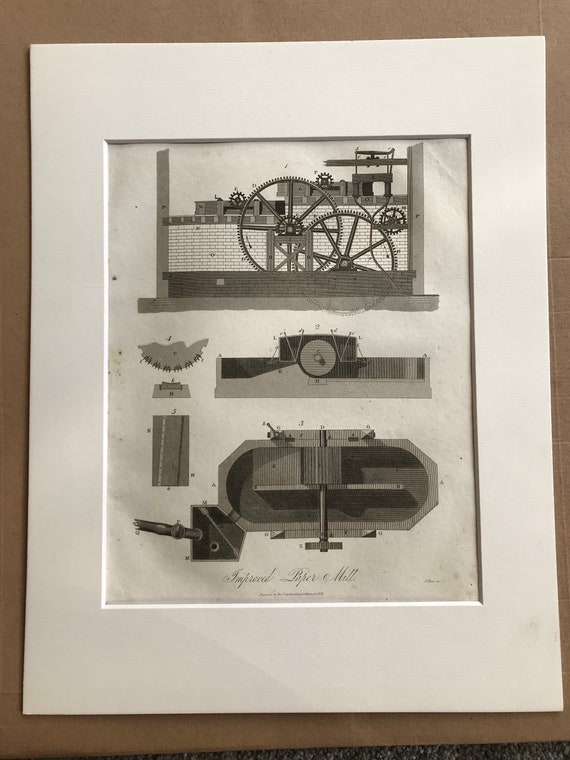The framed image presents a detailed, black-and-white illustration or blueprint of mechanical structures, divided into three distinct sections, each showcasing different mechanical components and designs. The top section illustrates a complex machinery setup featuring wheels, gears, and levers, all mounted on a brick base, indicative of a sophisticated mechanical assembly. The middle section focuses on circular elements, possibly wheels or gears, enriched with intricate detailing and numbering, suggesting a high degree of precision and technical design. The bottom section depicts an oval-shaped structure with internal compartments and external levers, resembling a floor plan or top view of a machine or building, complete with a propeller-like component. This meticulous drawing is encased in a white frame that contrasts with the detailed black ink sketches and is placed on a brown surface, likely a table or floor. Despite some blurriness that makes the signature at the bottom difficult to read, the overall bright setting and intricate details illuminate the mechanical artistry captured within the illustration.